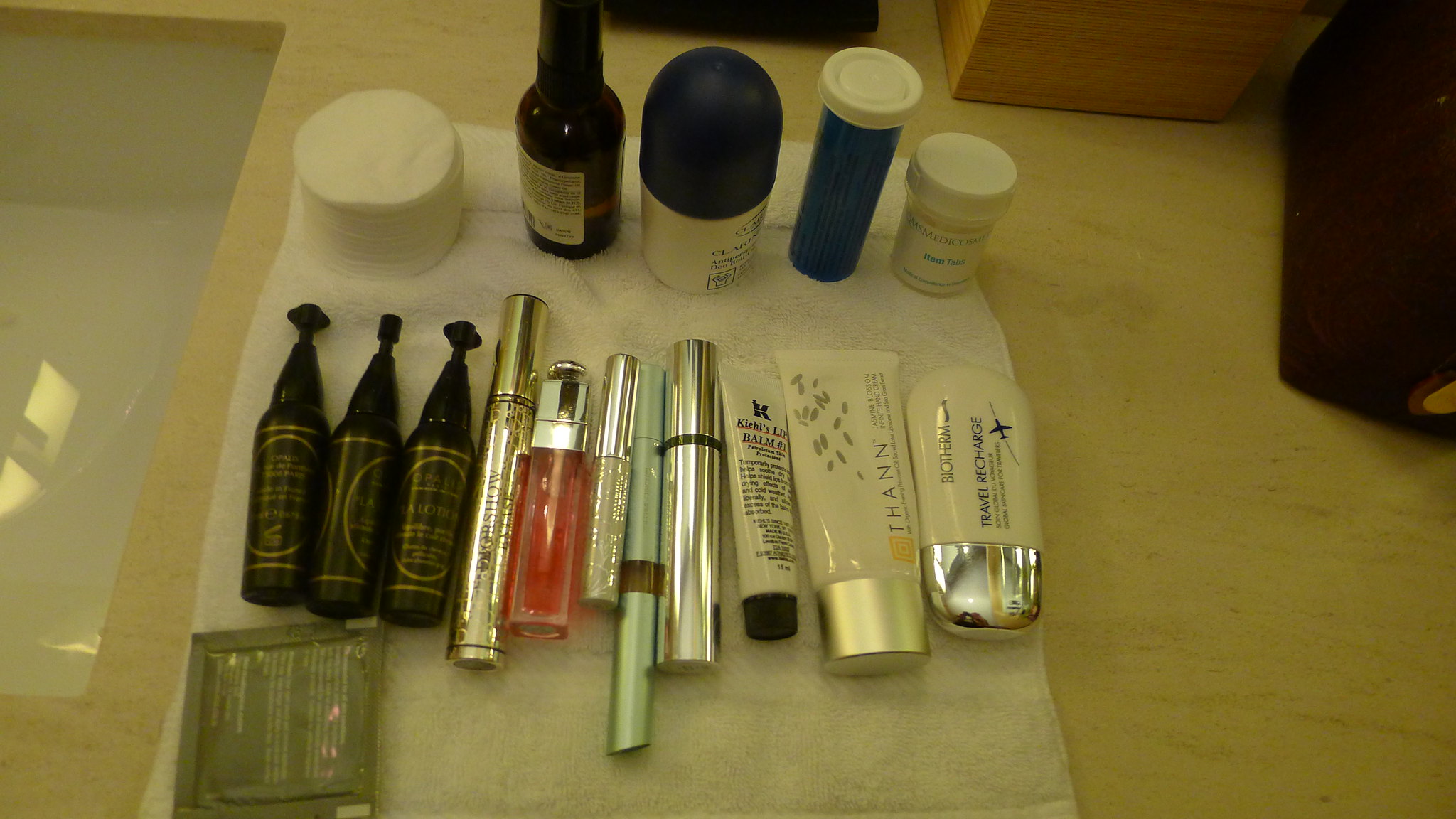The image features an assortment of various beauty products meticulously arranged on a buff-colored table or countertop. A neatly laid out washcloth forms the base of the display. To the left, a small, green pouch, likely containing moist towelettes, rests, hinting at its practicality. Prominently displayed are three small, dark bottles, the size of mini bottles, adorned with black lids and gold writing, exuding a sense of luxury. Beside them, a collection of makeup tubes, potentially comprising lipstick, eye paint, eyeliner, and mascara, stands ready for use. Additional makeup tubes of similar style accompany them, hinting at a broad selection. Completing the arrangement are a couple of prescription bottles, interspersed with a sizeable stack of cotton discs, essential tools for makeup removal. This carefully curated assortment reflects a comprehensive and organized beauty regimen.